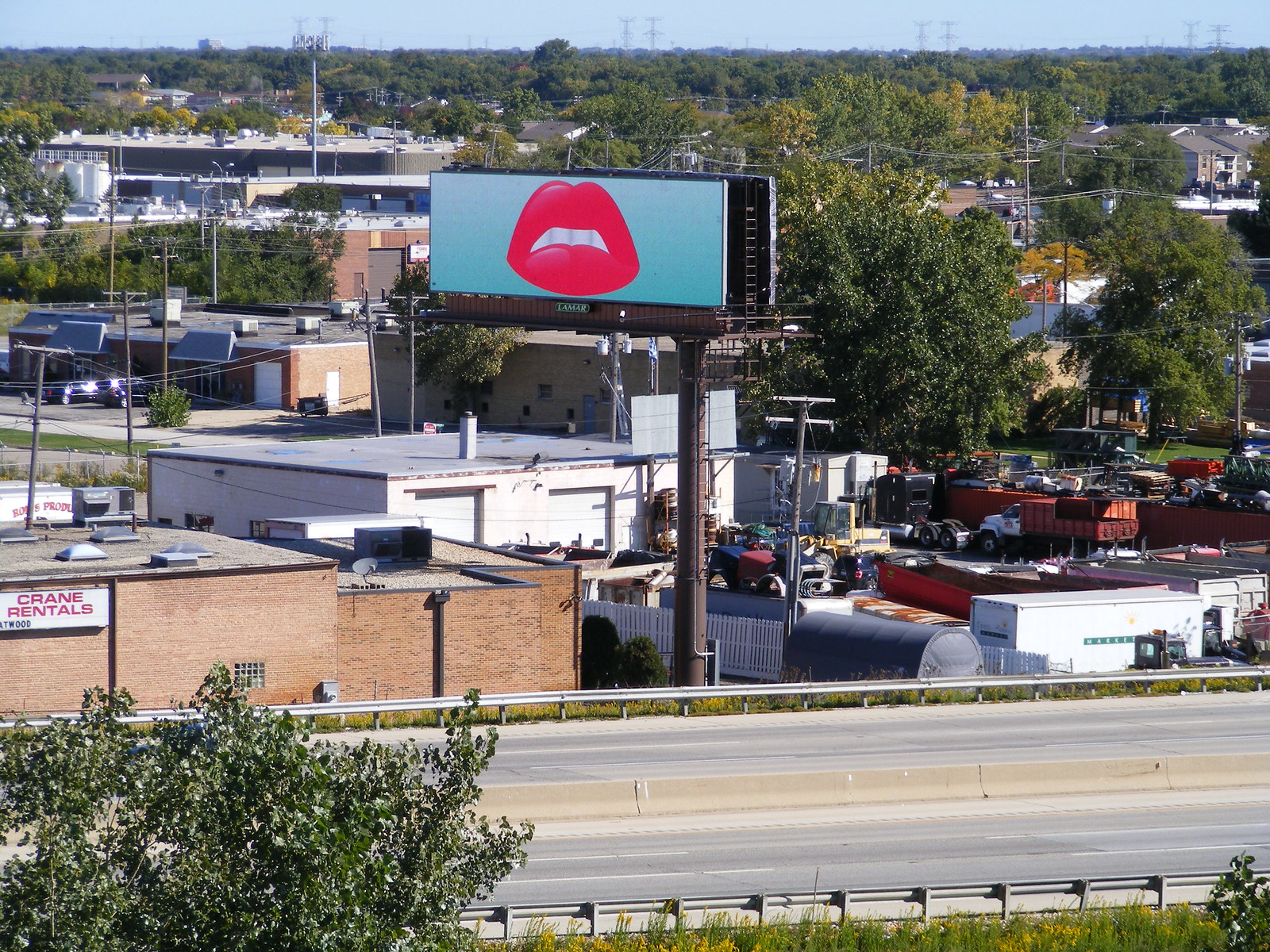In this realistic photograph taken from an elevated vantage point in a city, the foreground reveals a small patch of grass and the top of a tree protruding from it. Beyond the grass, two metal edges can be seen, likely marking the sides of a roadway. A stone median separates two roads. Following the roads, another metal strip is visible, leading to a larger expanse of grass that dips into what seems to be a hill.

Centered in the middle of the image stands a tall metal pole supporting a sign. The sign is light blue with a depiction of red lips frowning. In the background, numerous buildings are scattered among a lush array of trees, interspersed with a couple of tankers and cars. The skyline is filled with more trees, set against a backdrop of blue sky.